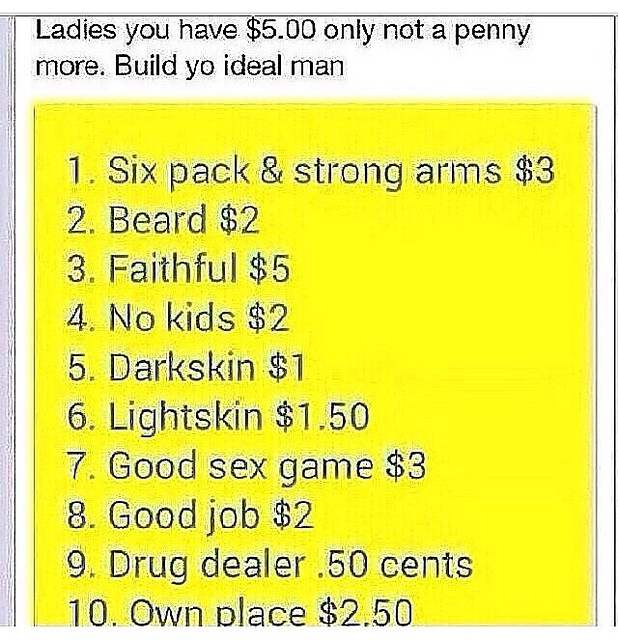The image appears to be a promotional poster or advertisement with a thick grey border, particularly noticeable on the left side. At the top of the poster, set against a white background, there's a bold black text that reads, "Ladies, you have $5, only not a penny more. Build yo ideal man." Below this, there is a prominent yellow box containing a list of 10 options in black text, each associated with a trait and its cost for building the ideal man: 

1. Six pack and strong arms, $3
2. Beard, $2
3. Faithful, $5
4. No kids, $2
5. Dark skin, $1
6. Light skin, $1.50
7. Good sex game, $3
8. Good job, $2
9. Drug dealer, $0.50
10. Own place, $2.50

This structured layout challenges women to select attributes that sum up to a total of no more than $5, emphasizing a playful take on preference prioritization through a simple, eye-catching design.